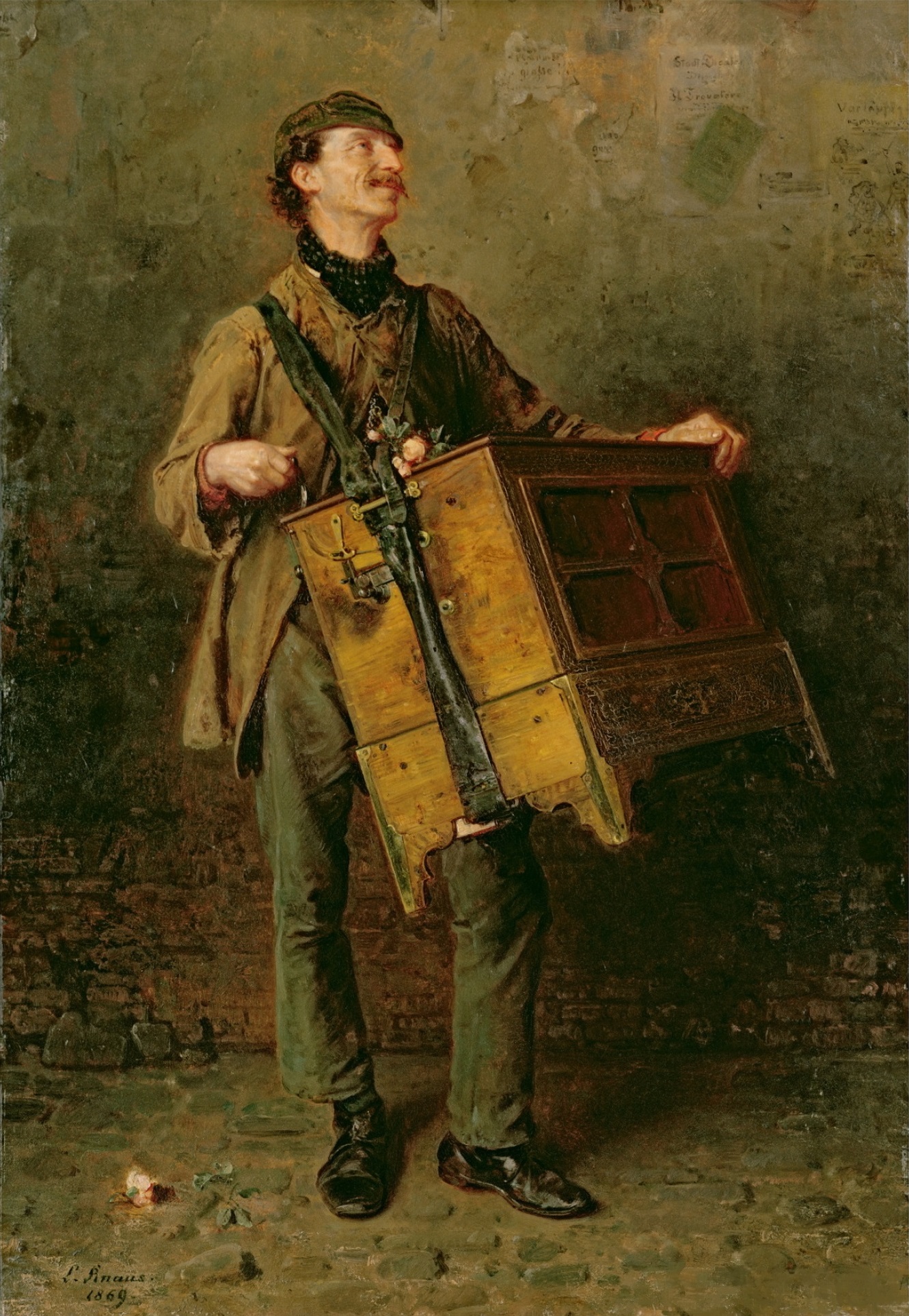This painting, signed by the artist in the lower left corner, depicts a street vendor who appears to specialize in music. The middle-aged man, likely in his forties, has fair skin and sports a brown mustache. He is attired in a wrinkled and worn brown jacket, gray pants, and black shoes. Wrapped around his neck is a black scarf, and his head is adorned with a scally cap.

He carries a large musical instrument—possibly a wind-up organ—suspended from a strap over his shoulders. His expression is one of contentment, as he smiles and looks upward to his right. The background features a red brick wall, aged and covered with moss, transitioning into a cement section. The man stands on a cobblestone sidewalk where a piece of litter is visible. The detailed artwork captures the texture of the ground and the backdrop, completing an evocative outdoor scene from a bygone era.